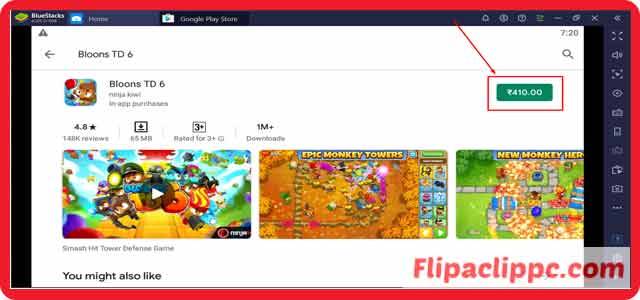This image appears to be a blurry screenshot of an online app store, likely the Google Play Store, featuring the game "Bloons TD 6." The image has a distinct red border, with a dark blue frame running across the top and down the right side, and a black frame on the left side. The central area within these borders is white.

In the top left corner, there is an indistinguishable green square, followed by a blue square with a home emblem and the text "Home," along with a reference to the "Google Play Store." Moving from right to left, there appear to be some icons or information that is not clear due to the blurriness.

Down the right side of the image, extending to the bottom, there are multiple icons. Within the white area of the image, the text "Paloons 2D" appears, and to its right, "720" is written with a search icon below it. There is a red rectangle with a white border on the right side, containing a green tab that reads "$410."

To the left of this rectangle, a red arrow points downwards towards a red triangle. Adjacent to this, there is a blurry circle or square with an image that is not clear. Below this, the text "Bloons TD 6" is visible, followed by its ratings, review count, and download information.

Towards the bottom, there are three additional game images displayed horizontally from left to right. In the bottom left corner, the text "You might also like" is visible, while the bottom right corner contains the text "Flip A Clip C.com."